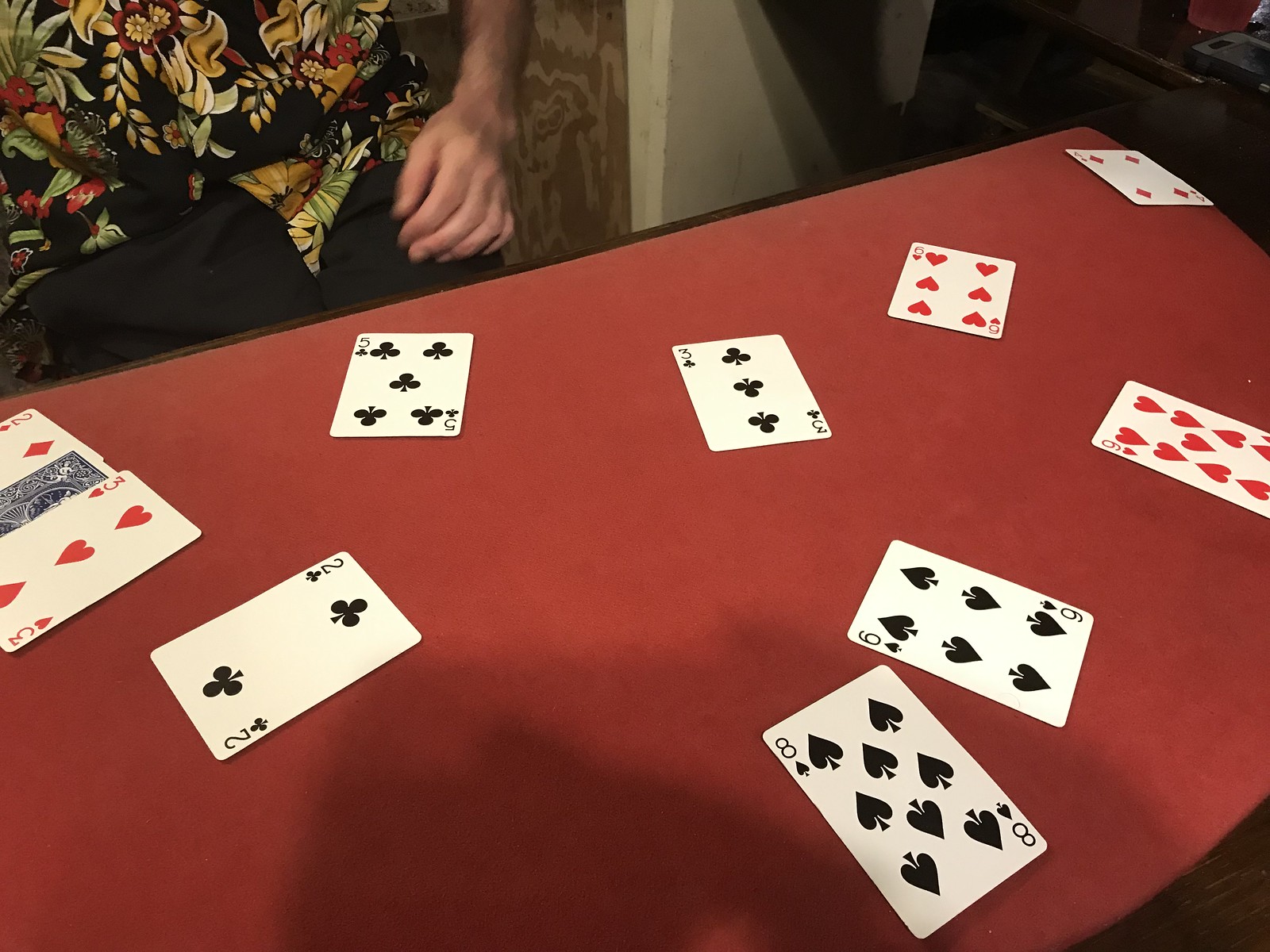The photograph captures an intense card game set on a vibrant red tabletop, which appears to be a felt or cloth material draped over a wooden brown table. Scattered haphazardly across the table are approximately a dozen playing cards, including the six and eight of spades, the two, five, and three of clubs, and a five of hearts. Among the mix, a diamond card is visible, though its specific rank remains unclear. Most of the cards lie independently, with only a trio of them touching each other.

Seated at the table is a Caucasian man, identifiable by his fair skin tone. He is clad in a striking floral shirt adorned with red and gold leaves, alongside floral buds, paired with black trousers. His left arm rests near the table's edge, partially revealing a neutral-toned wallpaper in the background, suggestive of a brown-colored wall adjacent to him. The overall scene presents a casual yet engaging atmosphere, with the scattered cards contributing to a sense of spontaneity.